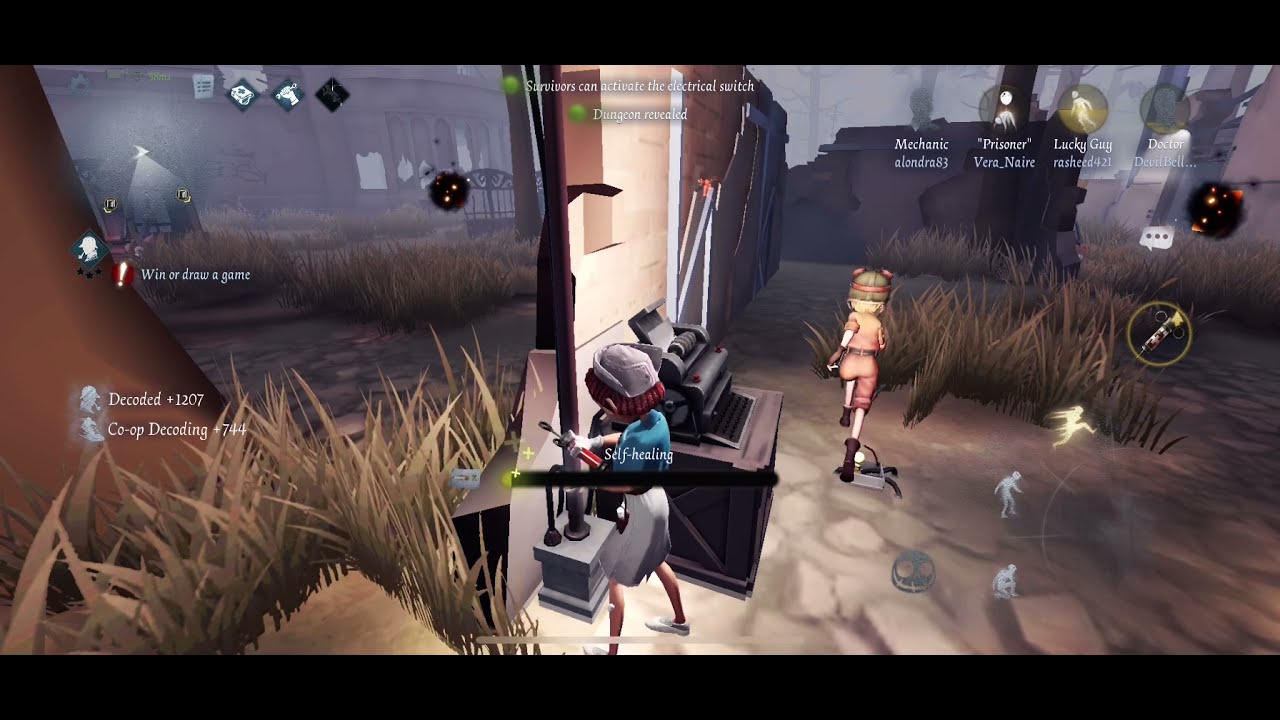This computer-generated image, seemingly from a video game, depicts a divided screen with detailed outdoor scenes set at night. On the left side, the terrain features a sprawling grass field extending towards a distant gate, with the text "decoded +1207, co-op decoding +744" superimposed in white. The backdrop includes a single standing wall of what appears to be a partially destroyed building, illuminated by a lamp, adding to the dreary atmosphere. Brown leaves and shrubs blend with the stone pavement, enhancing the ominous setting.

On the right side, two animated characters command attention. The character closest to the front is a young girl in a blue blouse, gray skirt, white shoes, and white cap. She is equipped with white gloves and holds a red and metal tool, standing next to a square object adorned with intricate gray machinery. Text reading "self-healing" and a progress bar float over her, indicating she is regaining power. Adjacent to her is another girl dressed in pink with a pink headband, pink shirt, pink shorts, and brown boots, donning a green military helmet. She appears to be running away from the camera across a muddy terrain interspersed with tall grass.

Topping the scene are four circles labeled "mechanic," "prisoner," "lucky guy," and "doctor," possibly indicating different character roles or statuses within the game. The overall ambiance is dark, hazy, and filled with a sense of desolation, capturing an intense moment in the game's narrative.